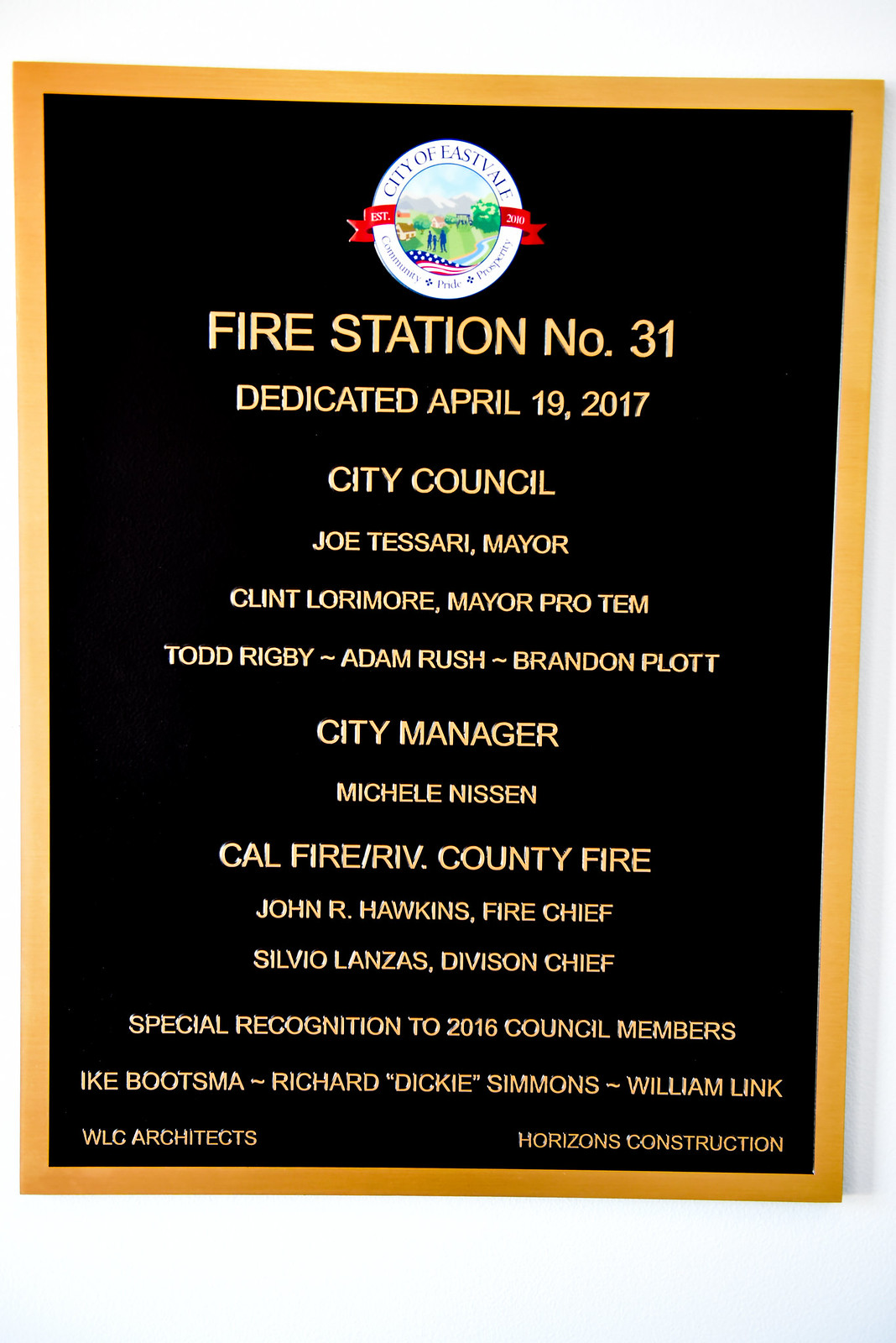The detailed description of the image shows a commemorative plaque for Fire Station Number 31 in the City of Eastville, dedicated on April 19th, 2017. The plaque is black with an orange rim, and the text is in a raised, metallic gold color resembling a plaque. At the top, within a circular segment, "City of Eastville" is written in white, accompanied by a scenic depiction with trees, people, an American flag, and a river. Below, the text lists the city council members in a line: Mayor Joe Tessari, Mayor Pro Tem Clint Lorimer, followed by council members Todd Rigby, Adam Rush, and Brandon Plot. It continues to name City Manager Michelle Nissen, and Cal Fire / RIV County Fire representatives: Fire Chief John R. Hawkins and Division Chief Silvio Lonza. There is also a special recognition to 2016 council members Ike Bootsma, Richard "Dickie" Simmons, and William Link. At the bottom, credit is given to WLC Architects and Horizons Construction. The plaque features aligned text, neatly organizing the dedication information and contributors involved.